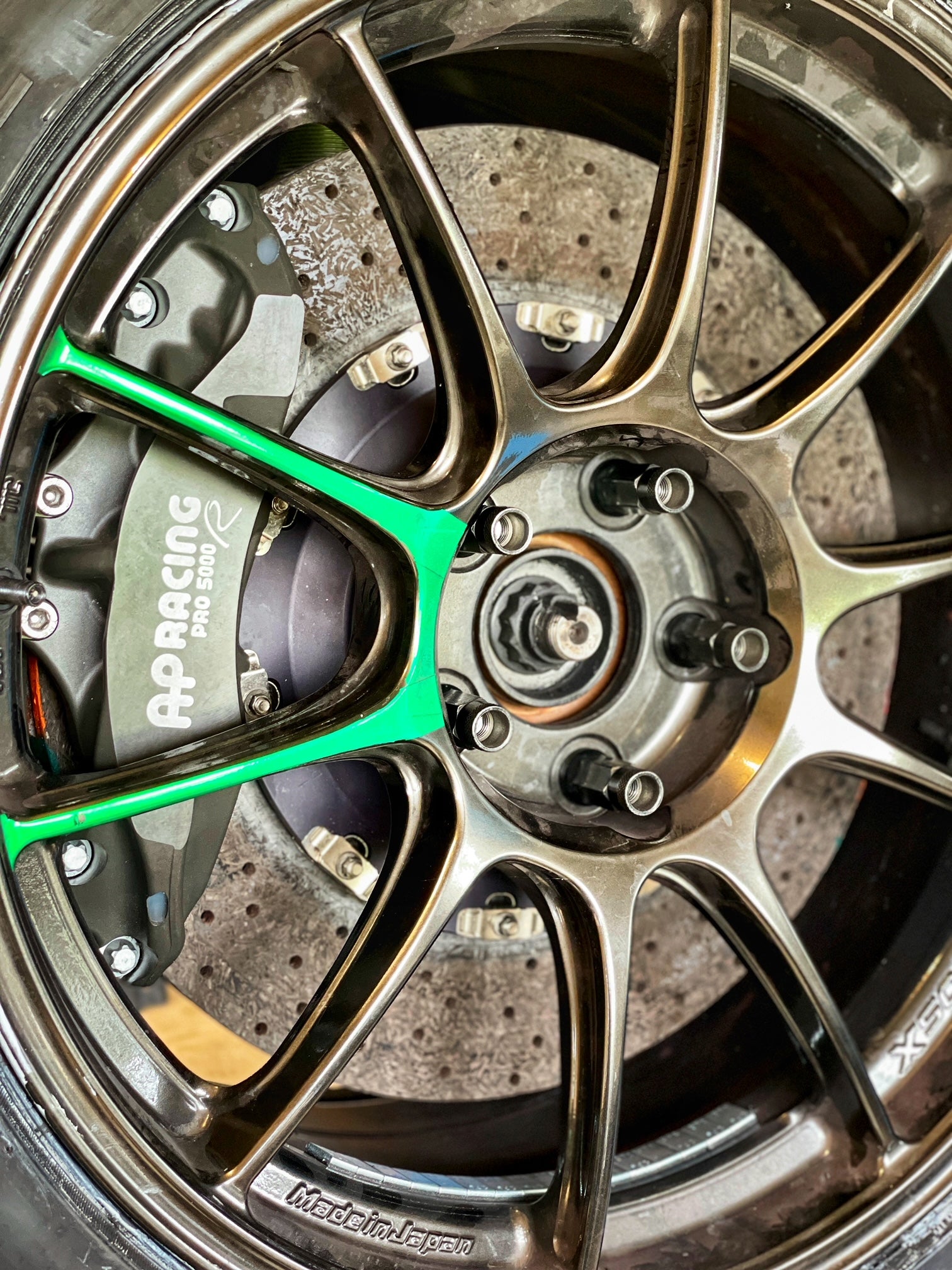The image showcases a rim for a racing tire, predominantly finished in a sleek satin black with a subtle sheen. Most of the spokes carry this satin black finish, except for two vibrant lime green spokes that stand out distinctly. Attached to the tire between these green spokes is a black metal label, extending inward from the outer edge of the rim. This label displays the words "AP Racing Pro 500" in white. Additionally, on the left side of the rim is a partial inscription, "AA Racing Pro 5000," contributing to the sense that this rim is designed for high-speed vehicles, possibly for a NASCAR racing car. There is another readable marking towards the bottom, "Made in Japan," and partially visible text on the right side that reads "X50." The rim itself appears hollow, offering a glimpse of the background through its structure, indicating a functional yet lightweight design suitable for competitive racing environments.